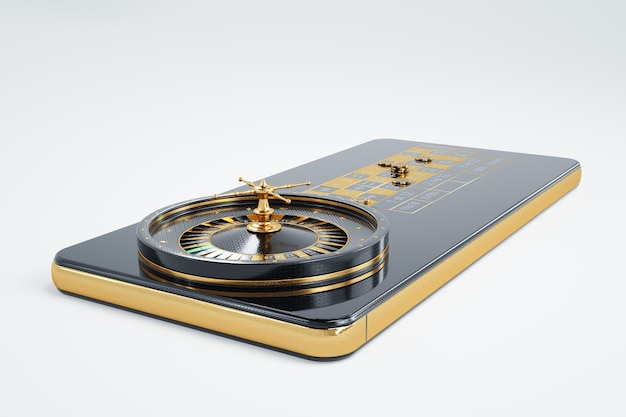This photograph depicts a unique product set against a white background. The central object, likely a miniature roulette wheel, is square and appears roughly the size of a phone or a small tablet. The edges are adorned with a gold trim, while the primary base color is black, creating a striking contrast. The wheel itself is detailed with black and gold elements and includes a gold center that likely spins. Surrounding the wheel are black and gold sections that resemble the layout of a roulette table, complete with spots where tiny black and gold poker chips – some possibly magnetic – can be placed. The intricacies of the roulette game are apparent, with gold accents scattered throughout and even a distinct green spoke among the wheel's features. Overall, the product is front and center in the image, showcasing its elaborate design and luxurious color scheme.